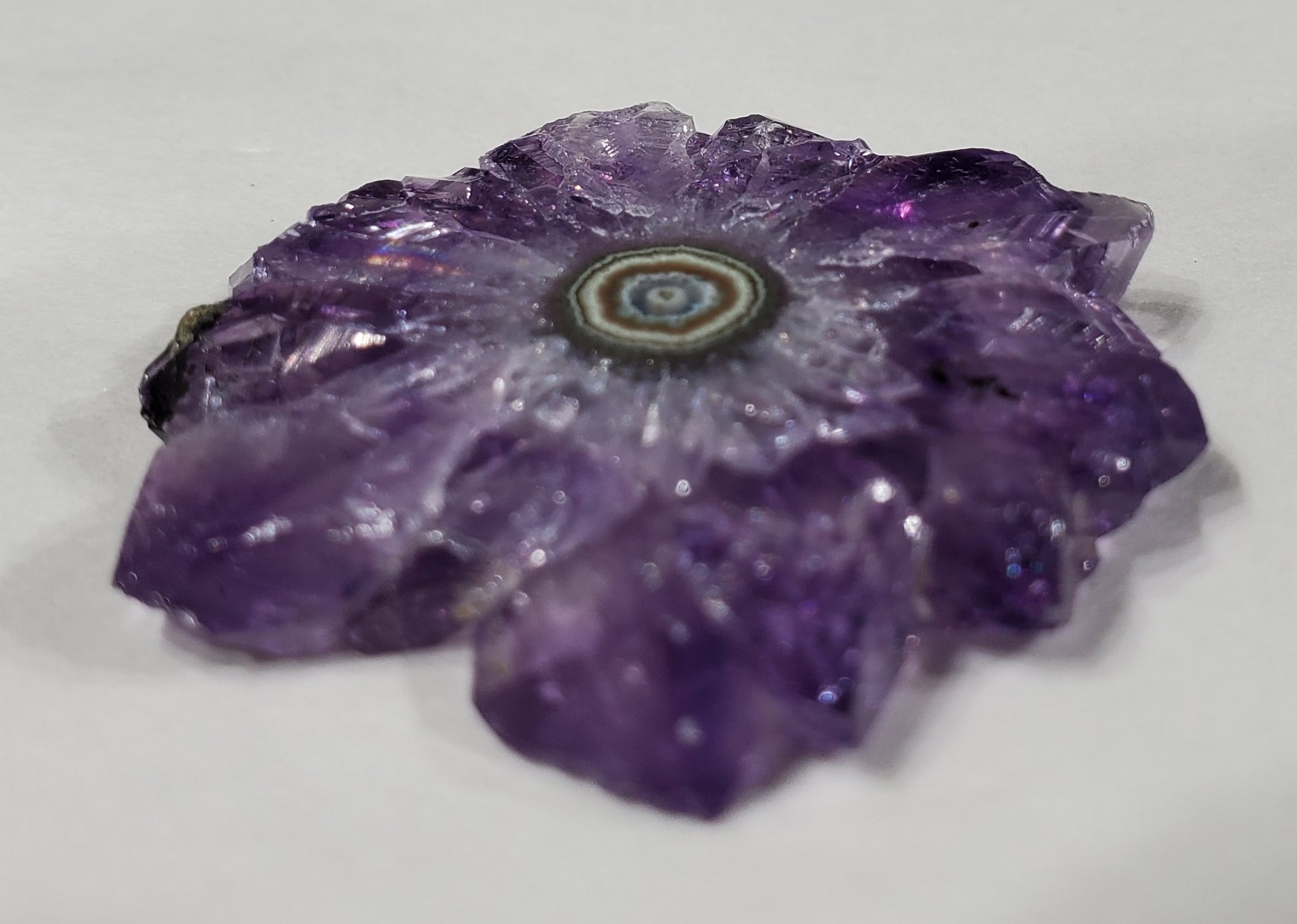This image captures a highly detailed and close-up view of a stunning, translucent, flower-shaped gemstone or crystal that has been cut in half to reveal its intricate inner structure. The outermost shell of the crystal is a striking dark purple, transitioning through gradients of purple towards the center. Surrounding this purple exterior are small white fragments that accentuate its petal-like shape. At the heart of the crystal, there is a captivating core that exhibits numerous concentric, ring-like layers, reminiscent of tree rings. These rings display a mesmerizing array of colors that include dark green, light green, orange, light blue, dark blue, and hints of white and reddish tones. The crystal is positioned on a white table, casting a noticeable shadow, suggesting a light source from above. The surface of the gemstone is highly reflective, further enhancing its lustrous and multi-colored appearance, making it shimmer with various hues as the light hits it.